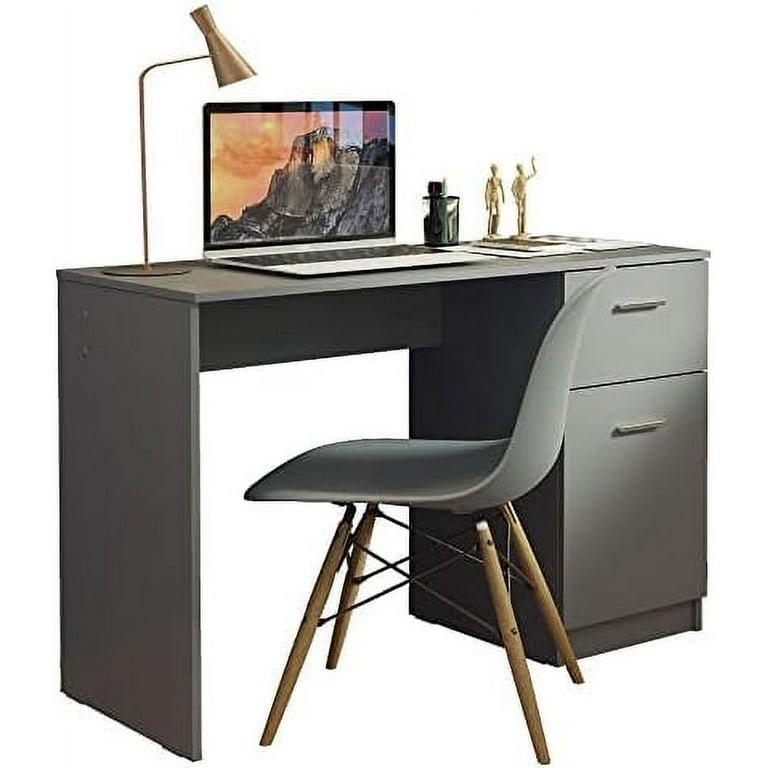The image showcases a minimalist, modern office setup against a completely white background. At the center is a gray desk around three and a half feet long and one and a half feet wide, constructed from flat pieces of gray wood. Positioned in front of the desk is a modern chair with a single-body design and brown wooden legs, lacking armrests. To the right of the desk are two drawers, with the bottom one being larger than the top. On top of the desk sits a sleek, metallic lamp with a design that arcs upward from the base and then bends at a 90-degree angle to shine downwards. An open laptop is placed on the desk, displaying an image that seems to be a mountain. Flanking the laptop are two small, gold-trimmed statues of people, one of which is raising its arm. Adjacent to the statues is a dark, indeterminate item. Additionally, some papers are scattered on the desk, adding to the realistic office ambiance. The entire scene has a crisp, clean aesthetic, typical for an advertisement or stock photo.